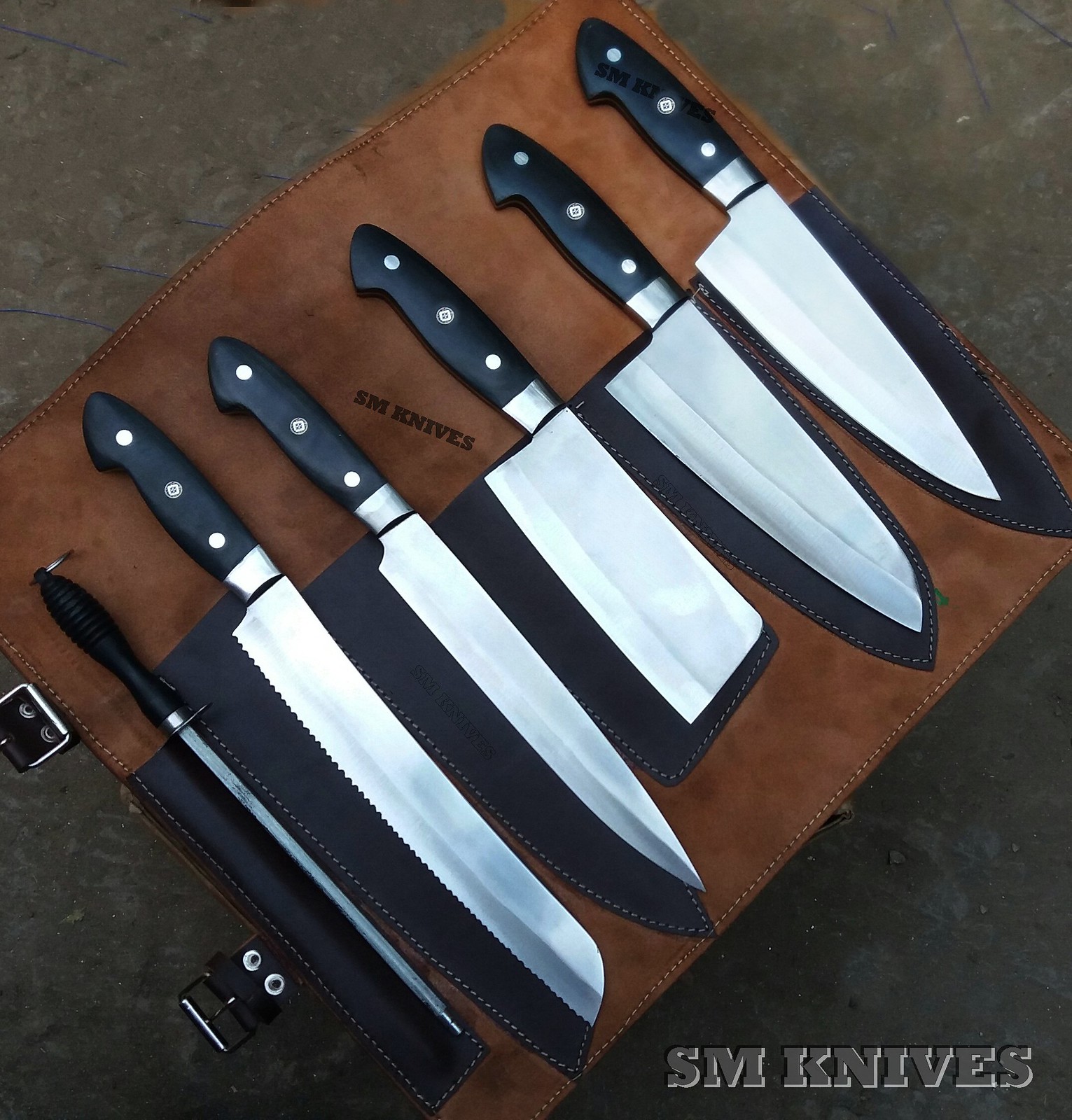This photograph features a meticulously arranged set of kitchen knives displayed on a dark grayish-brown surface that could be either concrete or marble. Lying diagonally across the surface is a brown leather roll-up pouch, complete with dark brown stitched sections designed to hold each knife securely. The pouch has a couple of buckles that allow it to be rolled up and clipped shut.

In total, there are six knives and one sharpening tool. Starting from the left, the layout includes a long, file-like sharpening tool, followed by a serrated blade, reminiscent of a bread knife. Next to the bread knife are two chef's knives with smooth blades, a cleaver with a weighted point, a standard meat knife, and at the end, a butcher knife. Each knife fits precisely into its designated section within the pouch.

In the bottom right-hand corner of the photograph, there is a bold watermark inscribed with "SM Knives." This same branding, "SM KNIVES," is also elegantly engraved on the leather pouch, adding a touch of authenticity and craftsmanship to the overall display. The background has a mottled brown and tan appearance, adding contrast and highlighting the array of knives laid out in the image.